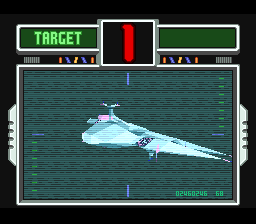The image is a close-up of a screen from what appears to be a video game, likely from the Star Fox series. The screen is framed by a black background with two silver or white handles extending outwards from each side. The top of the screen features a border with two green rectangles on either side of a black square outlined in silver. The left rectangle displays the word "Target" in light green letters, and the center black square contains a red number "1."

The main gameplay area is predominantly blue and green, resembling water, with a spaceship positioned centrally. This spaceship is all white, with two pointed ends extending to the left, and it slants downward from the middle-right to the left. At the bottom of the screen, numerical values "02460246" and "60" are displayed. 

On the right corner of the screen, a set of blue and green lines appear, with blue lines marking the center and green lines on both sides, creating a symmetrical pattern. To the left of the screen, similar lines appear in reverse order. These green lines are smaller than the blue lines. Additionally, there are multi-colored lines—red, blue, and orange—that seem to be wired down from the top section where "Target" is labeled. 

The spaceship and interface elements within this screen allude to a space combat environment, possibly engaging in a targeting session, characteristic of a spaceship in a video game setting.